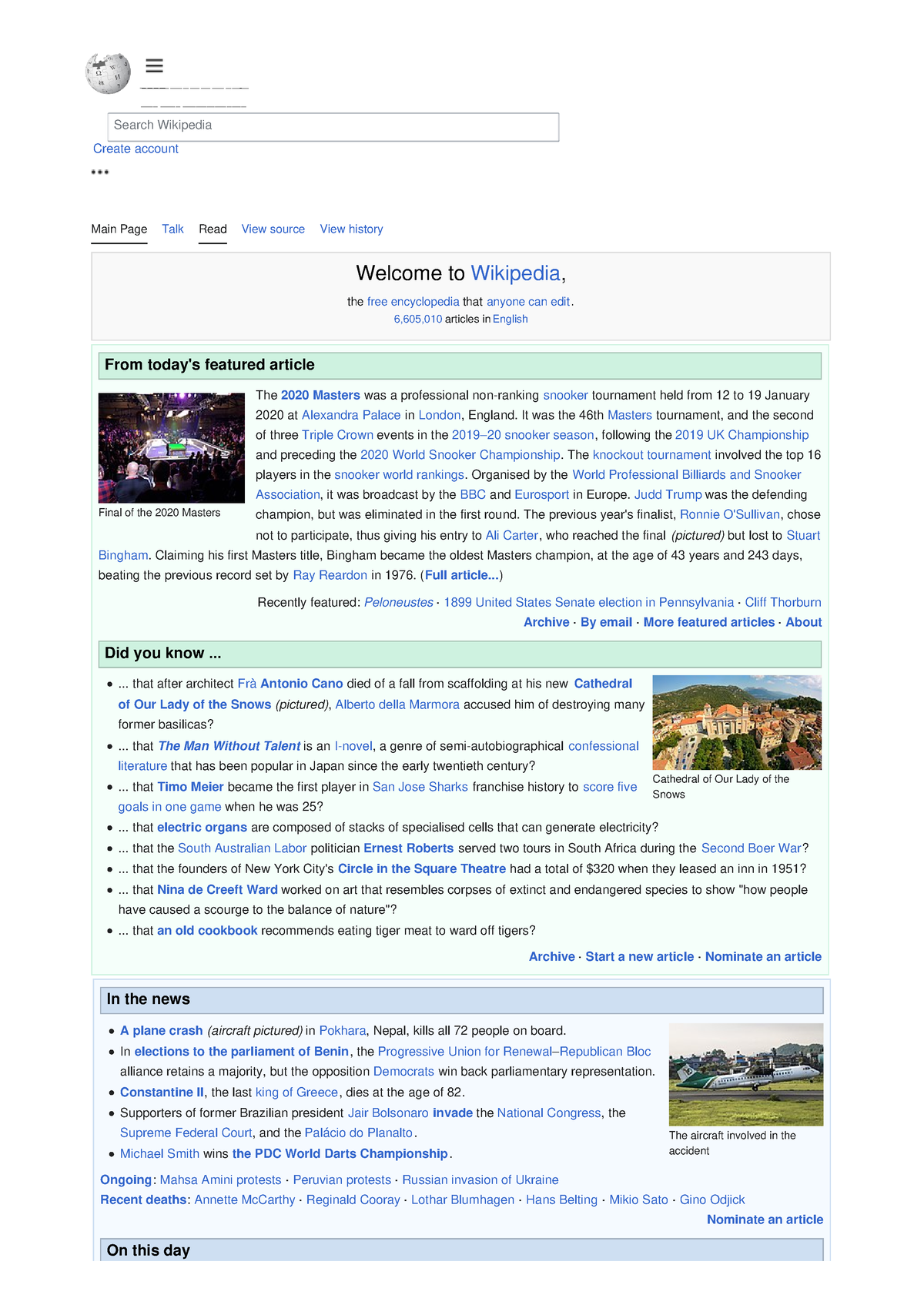Screenshot of a Wikipedia page detailing the 2020 Masters snooker tournament. The image prominently displays Wikipedia's interface with links for creating an account and navigating sections like the Main Page, Talk, Read, View Source, and View History. The page welcomes readers to Wikipedia, noting it is a free encyclopedia that anyone can edit and boasts 6,605,010 articles in English.

The featured article of the day discusses the 2020 Masters, a professional non-ranking snooker tournament held from January 12 to 19, 2020, at Alexandra Palace in London, England. This event marked the 46th edition of the Masters and was the second of three Triple Crown events for the 2019-20 snooker season, positioned between the 2019 UK Championship and the forthcoming 2020 World Snooker Championship.

The tournament was a knockout event featuring the top 16 players in the snooker world rankings, organized by the World Professional Billiards and Snooker Association. Broadcasting was covered by European networks including the Big Black Caulk and Eurosport.

Notably, Judd Trump, the defending champion, was eliminated in the first round, an unexpected result given his status. Additionally, the runner-up from the previous year, Ronnie O'Sullivan, opted not to participate, passing his spot to Ali Carter. Carter advanced to the final but ultimately lost to Stuart Bingham.

The detailed description also mentions a query about "snooker," indicating a possible side note or curiosity about the sport for readers unfamiliar with it.